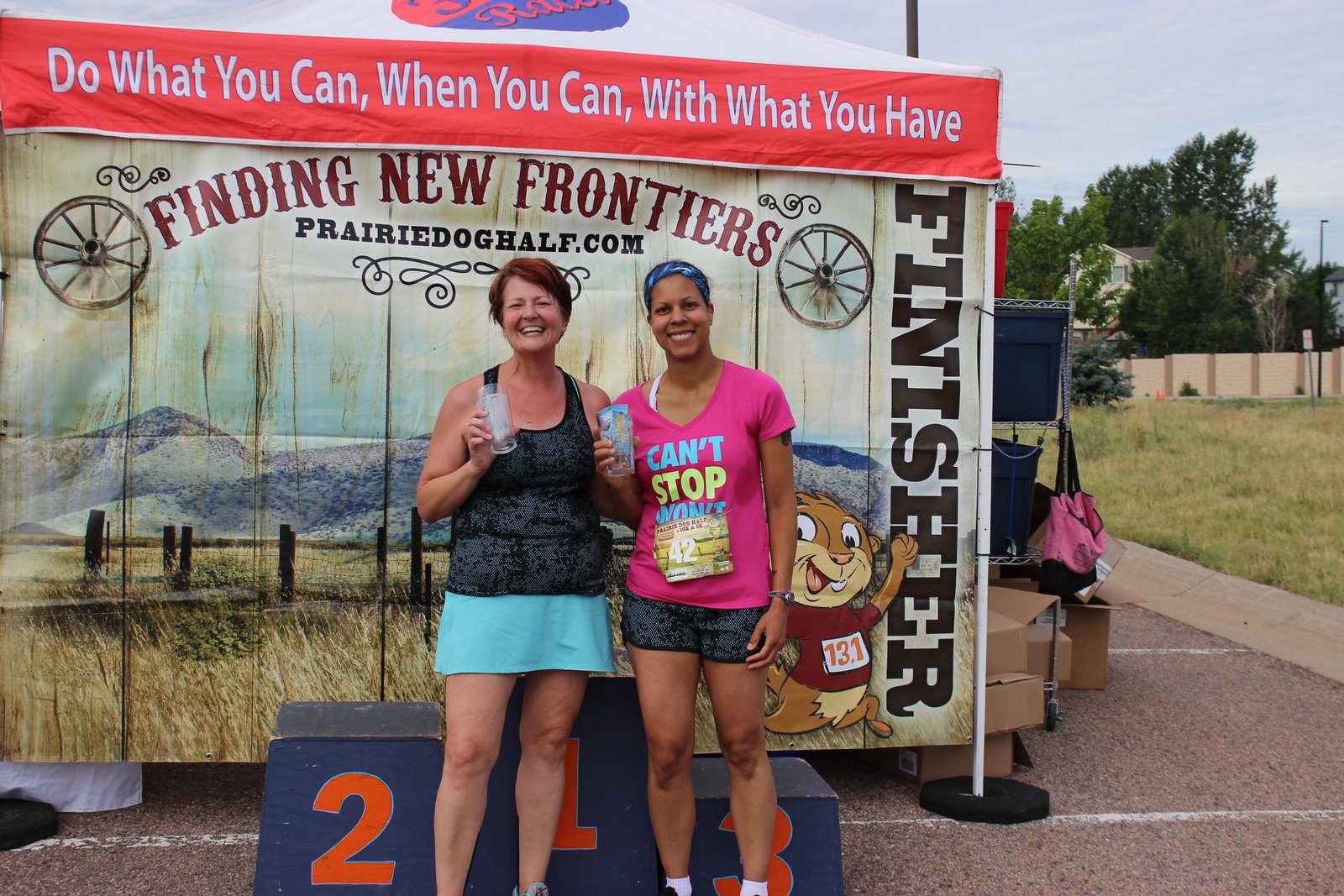The image depicts an outdoor scene featuring two women standing in front of a blue podium marked with the numbers 1, 2, and 3 in orange paint. In the background, there is a large tent adorned with an advertisement for PrairieDogHalf.com, featuring the slogan "Finding New Frontiers" and the word "FINISHER" running vertically down the right side. The tent also depicts a prairie dog wearing a number 131 jersey. The woman on the right, dressed in a pink "Can’t Stop, Won’t Stop" t-shirt partially covered by a race bib numbered 42, and sporting a blue bandana and black shorts, seems to have participated in a race. The woman on the left is wearing a black sleeveless tank top paired with a short blue skirt. Both women are holding small cups, possibly for drinking. Surrounding them, the setting includes trees, a grassy area, a brown fence, and some blue sand dunes, contributing to the natural, serene ambiance of the scene. Additionally, an orange banner at the top of the tent reads, "Do what you can, when you can, with what you have."